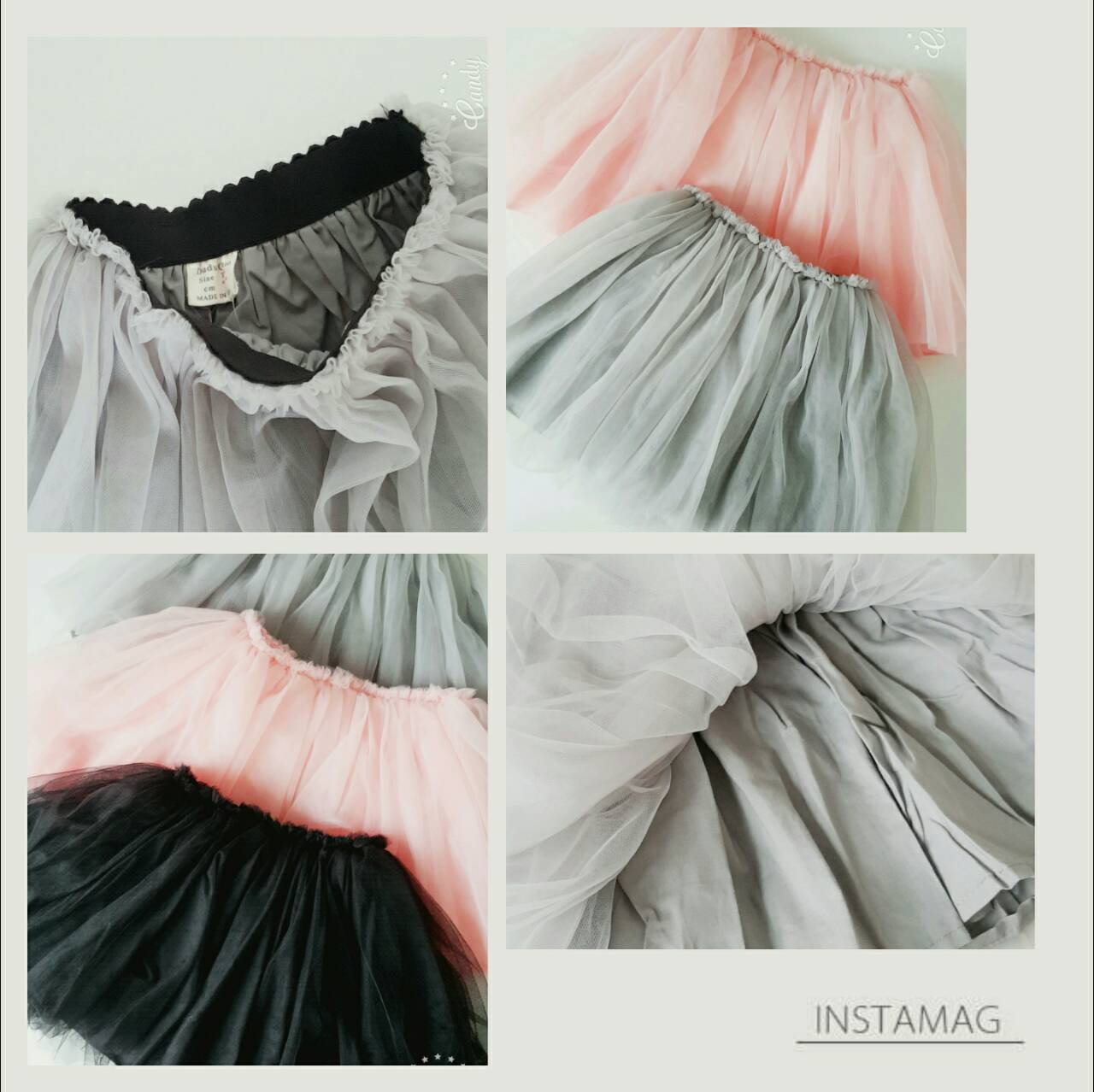The image is a collage consisting of four smaller photos arranged in a grid against a steel gray background, separated by white lines. In the bottom right corner, the word "Instamag" is underlined. The collage showcases various skirts, all appearing to be in tall, tutu-like styles roughly between sizes 5 and 7, with a mix of black, gray, and pink colors. 

1. The top left quadrant features a partially see-through black and gray skirt with a dark brown pleated waistband, partially pulled down to show its inside, which is black and tagged.
2. The top right quadrant displays a gray skirt partially covered by a pink skirt, revealing layers of tulle.
3. The bottom left quadrant combines a gray skirt, a pink skirt, and a black skirt, stacked in layers, highlighting their tulle structures.
4. The bottom right quadrant offers a close-up of a gray skirt with a frilly white overlay, showing detailed netting and pleating. 

Each photograph contributes to a detailed and tactile understanding of the skirts, emphasizing their colors, layering, and textures.